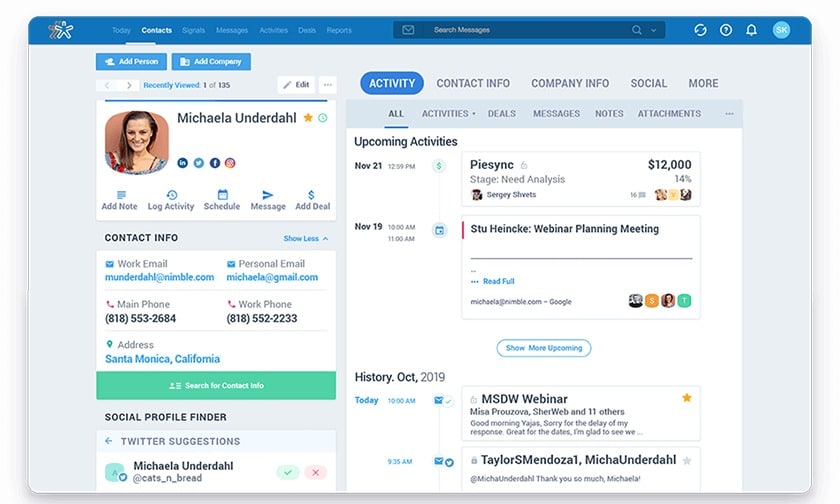This image is a meticulously detailed screenshot taken from either a website, mobile phone, or tablet. Prominently displayed is the profile of Michaela Underdahl. Her profile picture captures her head and shoulders, dressed in a striking red and blue floral dress with a red strap. Adjacent to her picture are four social media icons for LinkedIn, Twitter, Facebook, and Instagram.

Beneath her profile picture, a set of five icons represents various functionalities: ad note, blog activity, schedule, message, and ad deal. Following this is a "Contact Info" section, detailing both work and personal emails, main phone, work phone, and lists her location as Santa Monica, California. Below this information, a vibrant green call-to-action bar encourages users to "search for contact info." 

Further down, there is a "Social Profile Finder" section, showcasing Twitter suggestions. On the right-hand side, the interface is neatly divided into five main sections: Activity, Contact Info, Company Info, Social, and More. The "Activity" section is highlighted, revealing subheadings such as all activities, deals, messages, notes, and attachments. This section comprehensively displays all upcoming activities and historical data related to Michaela Underdahl.